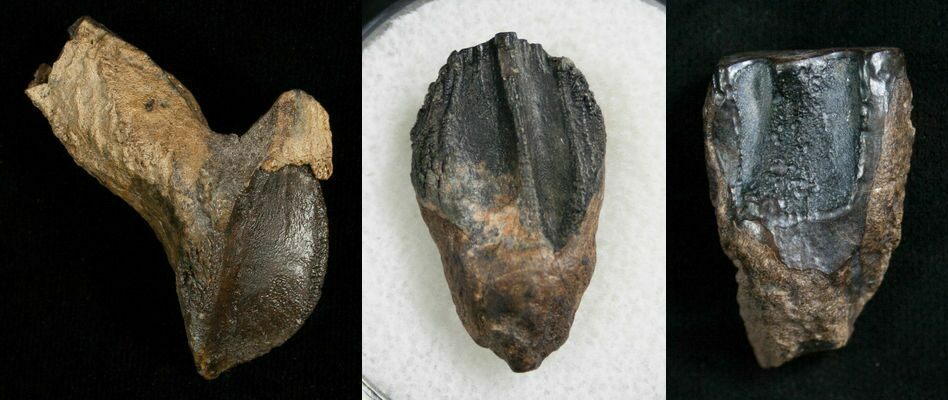The image displays three side-by-side photographs, each showcasing a distinct yet similar artifact, likely of ancient origin. The first artifact, set against a black backdrop, appears to be chiseled from stone, with a predominantly dark coloration that transitions to a lighter stone texture towards the bottom. It has a rough, arrowhead-like shape with curves and a pointed tip. The central artifact, displayed on a white background, resembles a fossilized footprint or hoof print, characterized by an oval shape and noticeable ridges. Its coloration transitions from grayish-black at the top to brown at the bottom. The third artifact, also set on a black backdrop, exhibits an irregular shape with an indentation at the center. It features a rough texture, with significant black areas on the top and center portions, suggesting it could be a piece of stone or sediment. Despite their varied appearances, the three artifacts share a rough texture and distinguished shapes, hinting that they might be related or part of the same collection.